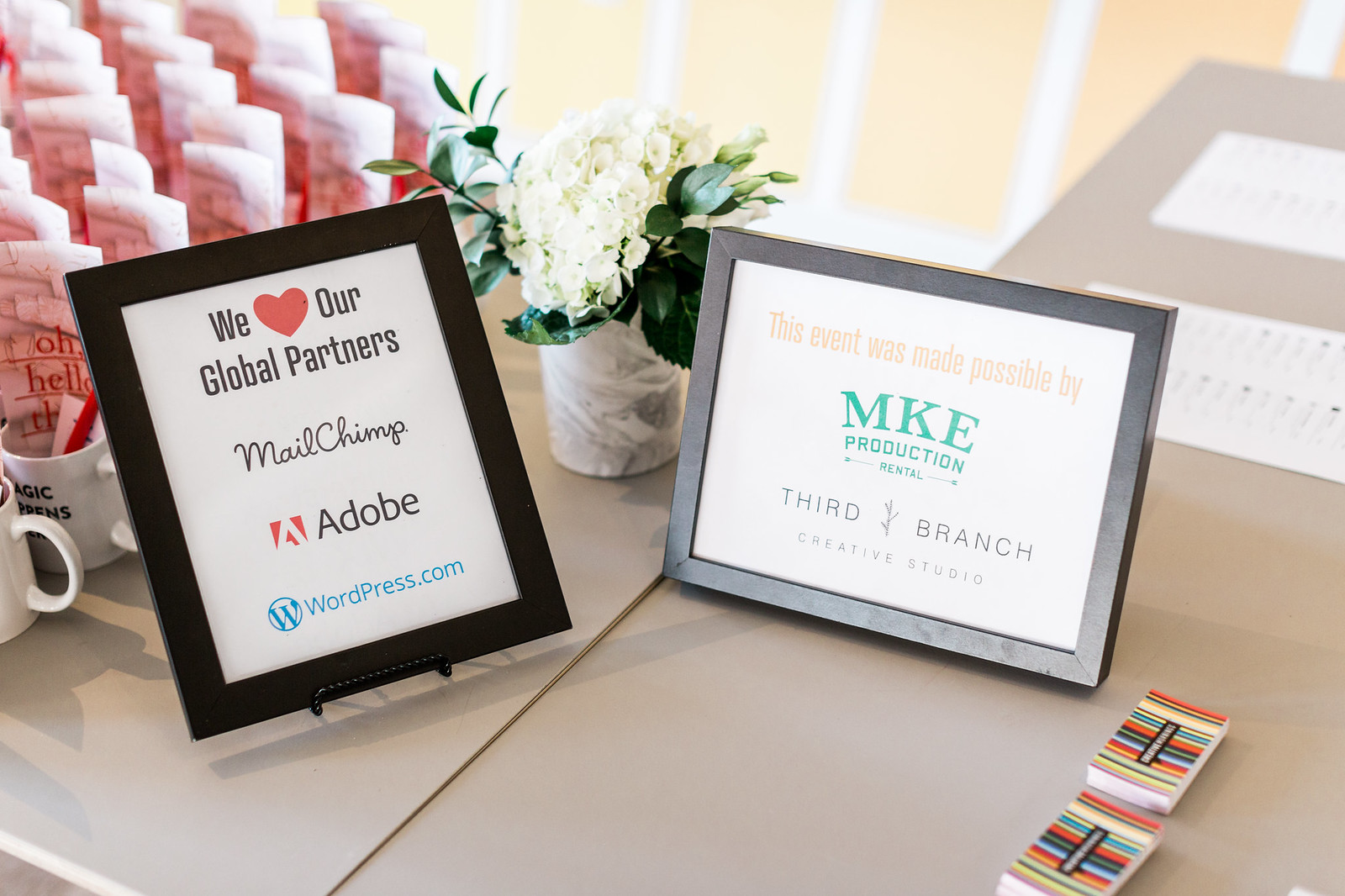The image depicts a well-organized, L-shaped brown desk set up indoors during what appears to be a conference. Prominently centered on the desk are two framed signs: one reading "We Heart Our Global Partners, MailChimp, Adobe, WordPress.com," and the other stating, "This event was made possible by MKE Production Rental, 3rd Branch Creative Studio." On the left side of the desk, there are several coffee mugs filled with papers and pens, accompanied by stacks of rainbow-striped business cards. A vase containing white flowers with green leaves stands in the middle, adding a touch of elegance. The image features a variety of colors including yellow, white, gray, green, pink, orange, red, blue, tan, light blue, and the setting indicates that the event is taking place in the middle of the day.